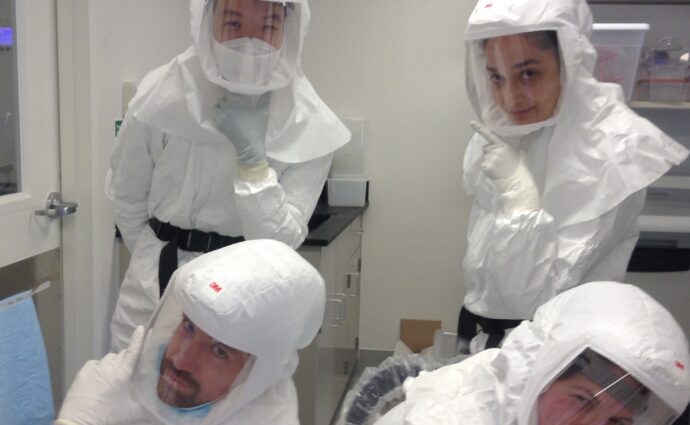In this image, four individuals are dressed in white hazmat suits complete with clear face shields, gloves, and black belts. They appear to be medical or lab professionals situated in a highly sterile, white room. The room features white walls, metallic door hardware, a black tiled countertop, shelves, and a silver sink or countertop. 

The group consists of two men and two women, all seemingly enjoying the moment with visible smiles and jovial expressions beneath their face shields. The man in the lower left corner has a beard and is gazing upwards with a sheepish grin. To his right, another man, possibly of Asian descent, appears partially out of frame, showing only his eyes which are squinting in amusement. A woman with black hair and black eyebrows stands in the upper right, pointing playfully towards the upper left side of the image. Another woman, partially obscured in the lower right corner, is looking down and to the right.

Their playful demeanor combined with the high level of protective gear and the clinical setting suggest they are taking a moment of levity in what is likely a serious work environment.